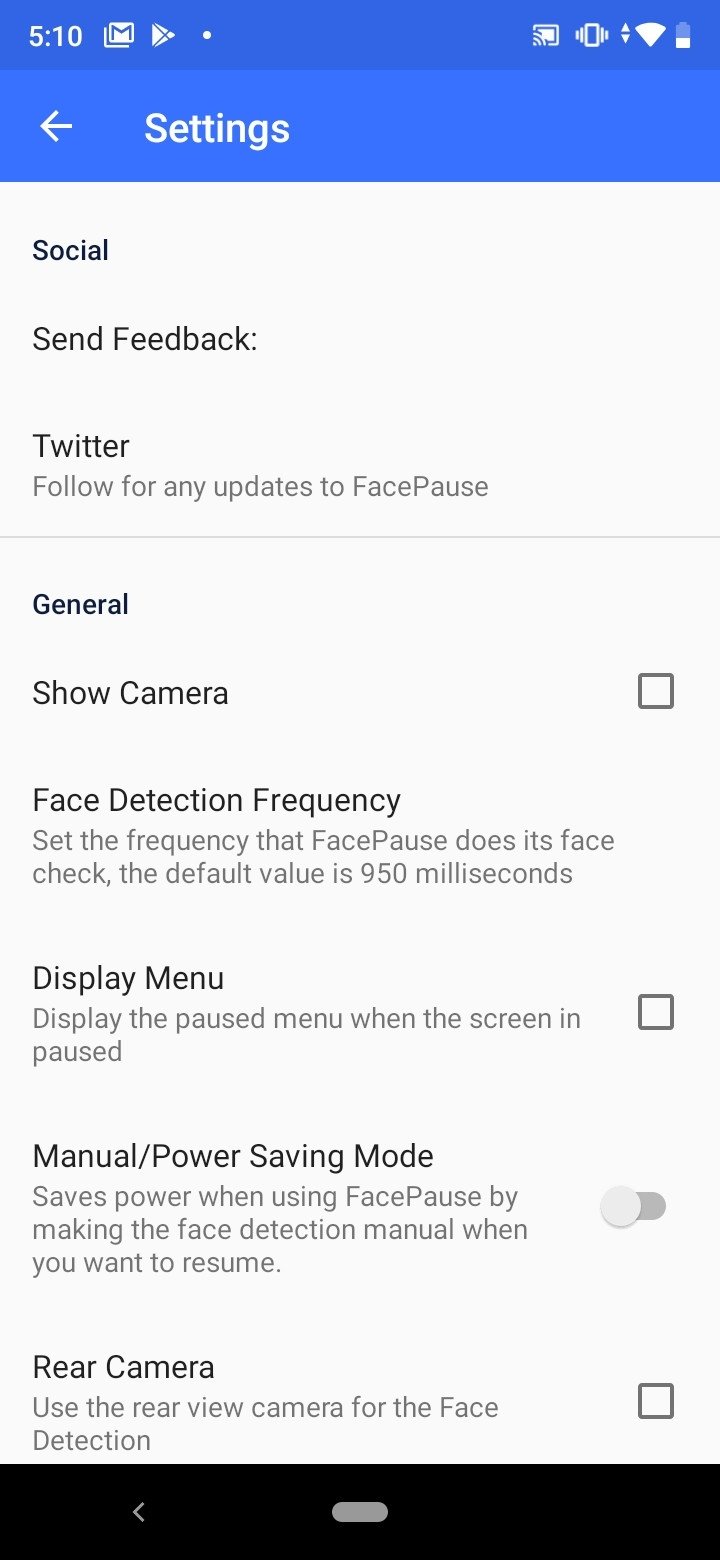This image is a detailed screenshot of a smartphone settings page with a white background. The top border is blue, where the time is displayed as "5:10" in white on the left side. To the right, small icons for email, a battery at approximately one-third charge, Wi-Fi, and a muted phone symbol are visible. Directly beneath this top section, there is a lighter blue header with the word "Settings" in white and a left-pointing white arrow.

The settings page itself is divided into sections. The first section, titled "Social," includes an option to "Send Feedback," accompanied by information about following updates for an app named "FacePause" on Twitter, with "FacePause" indicated as one word and an initial capital 'P' for "Pause." This section is separated by a thin horizontal line.

The next section is labeled "General" and contains various options such as "Show Camera," "Face Detection," "Frequency," "Display Menu," "Manual Power/Power Saving Mode," and "Rear Camera." Each option is followed by a brief description and a corresponding gray checkbox on the right side for activation.

The bottom border of the page is black, providing a clear end to the settings options listed. The overall layout is clean and systematically organized for easy navigation.